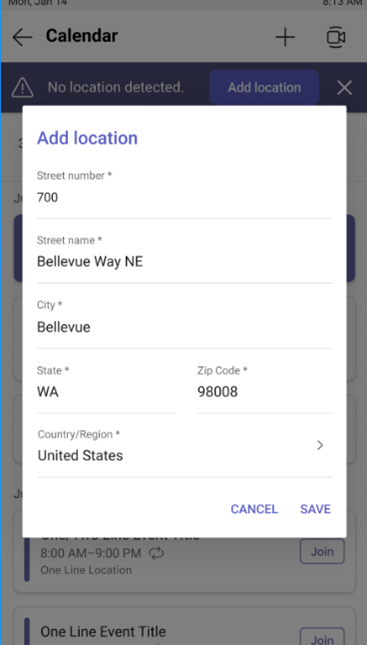This image is a partial screenshot of a smartphone's interface, specifically showing the status bar at the top, which displays the date as Monday, January 14th, and the time at approximately 8:13 a.m. The phone is currently open to a calendar application for event planning, where an "Add Location" pop-up is prominently displayed on the screen. This pop-up is centered against a white background with "Add Location" written in blue font at the top and fields for entering an address. The pre-filled fields include: street number "700", street name "Bellevue Way", city "Bellevue", state "Washington", ZIP code "98008", and country/region "United States". Below these fields, there are two buttons labeled "Cancel" and "Save".

Partially visible behind this pop-up is an error banner located under the main calendar header, which states "No Location Detected" and features an "Add Location" button and a "Close" button next to it. Slightly obscured behind the pop-up are other calendar entries and events, which are indistinct and not clearly readable. The overall impression is that the user is trying to add a location to a calendar event but has encountered an issue that is being addressed via the pop-up interface.